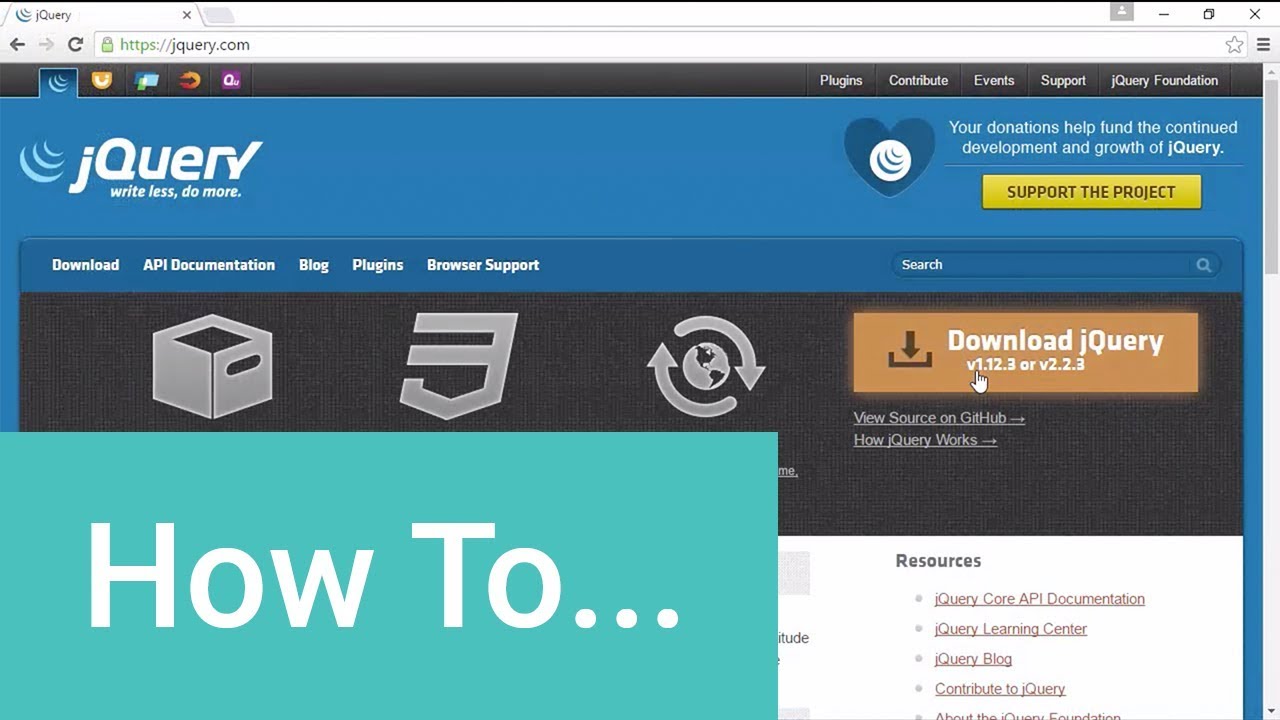This is a detailed screenshot of the jQuery website open in a web browser on a desktop PC. At the top, there's a white address bar displaying the URL: https://jquerv.com. Below the address bar, a black navigation menu features clickable options. The first option is selected, while others, listed in white font, include "Plugins," "Contribute," "Events," "Support," and "jQuery Foundation."

Beneath the navigation menu, a prominent blue banner spans the width of the screen. On the left side of the banner, the jQuery logo is displayed in white, consisting of three circular white lines symbolizing movement, along with the tagline "jQuery, Write Less, Do More." On the far right side of the banner, a white text message reads, "Your donations help fund the continued development and growth of jQuery." To the left of this message, a darker blue heart icon features the same three circular lines, reinforcing the brand's identity. The screenshot captures the professional and user-friendly design of the jQuery website, emphasizing both its functionality and its call to action for community support.